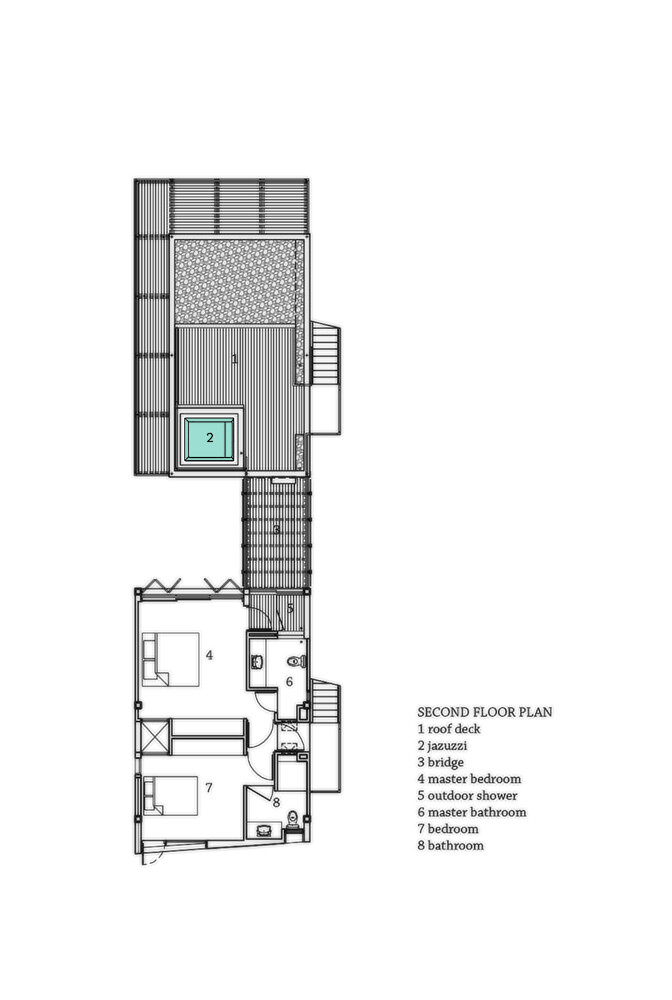This detailed blueprint illustrates the layout of a home's second floor. In the bottom right corner, the caption "SECOND FLOOR PLAN" is prominently displayed in all caps, alongside a legend. The diagram features two bedrooms, each with an en suite bathroom, situated towards the middle and lower part of the image. To the top of the blueprint, a spacious roof deck (labeled 1) is connected to a larger deck area (labeled 2 as Jacuzzi), highlighted in light teal to represent the water in the hot tub. Adjacent to this setup, a bridge (labeled 3) links the roof deck to the master bedroom (labeled 4) below. Furthermore, an outdoor shower (labeled 5) can be seen near the master bedroom, leading into the master bathroom (labeled 6). Besides the master suite, there is another bedroom (labeled 7) with its corresponding bathroom (labeled 8). The entire blueprint is meticulously drawn with fine black lines, emphasizing each room and feature's distinct placement and function.